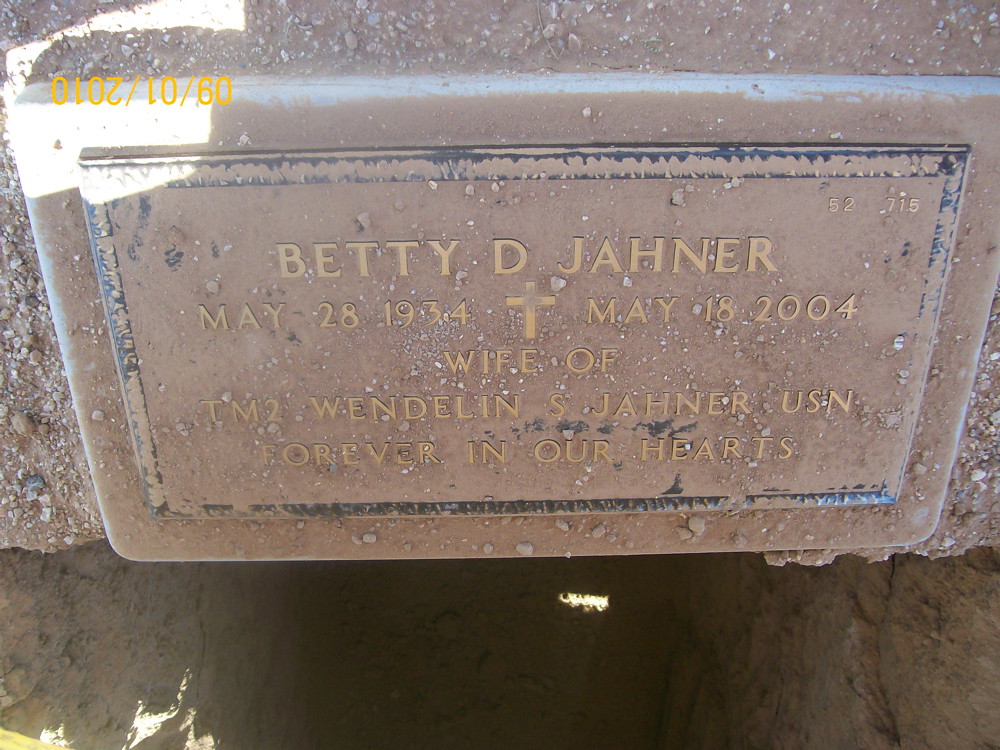The image depicts a flat, weathered gravestone with a brownish-beige hue, perhaps once white but now worn and covered in dirt and stones. The gravestone belongs to Betty D. Johnner, born May 28th, 1934, and passed away on May 18th, 2004, inscribed with "wife of TM2 Wendland S. Johnner, USN, forever in our hearts," accompanied by a small cross. Positioned above an empty hole, this gravestone appears partially buried and possibly in the process of being relocated or repositioned within the cemetery. The mud-covered plaque suggests it might have been recently uncovered or detached. Nearby, an additional date, 0901 2010, is visible, possibly indicating a related activity or event.